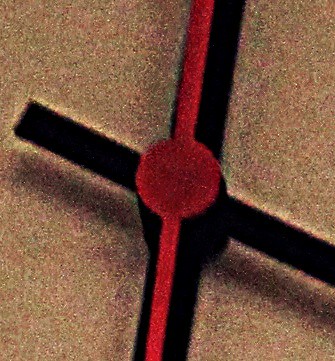The image depicts a red cylindrical valve positioned horizontally across the center, with a metal pole passing through its core. The valve features two prominent, red, column-like extensions on either side. The pole, emerging from the left and extending to the right, slopes slightly downwards as it traverses the valve. The photograph has a grainy texture, indicating a low resolution, and the background consists of a brownish surface, possibly a workbench or similar setting.